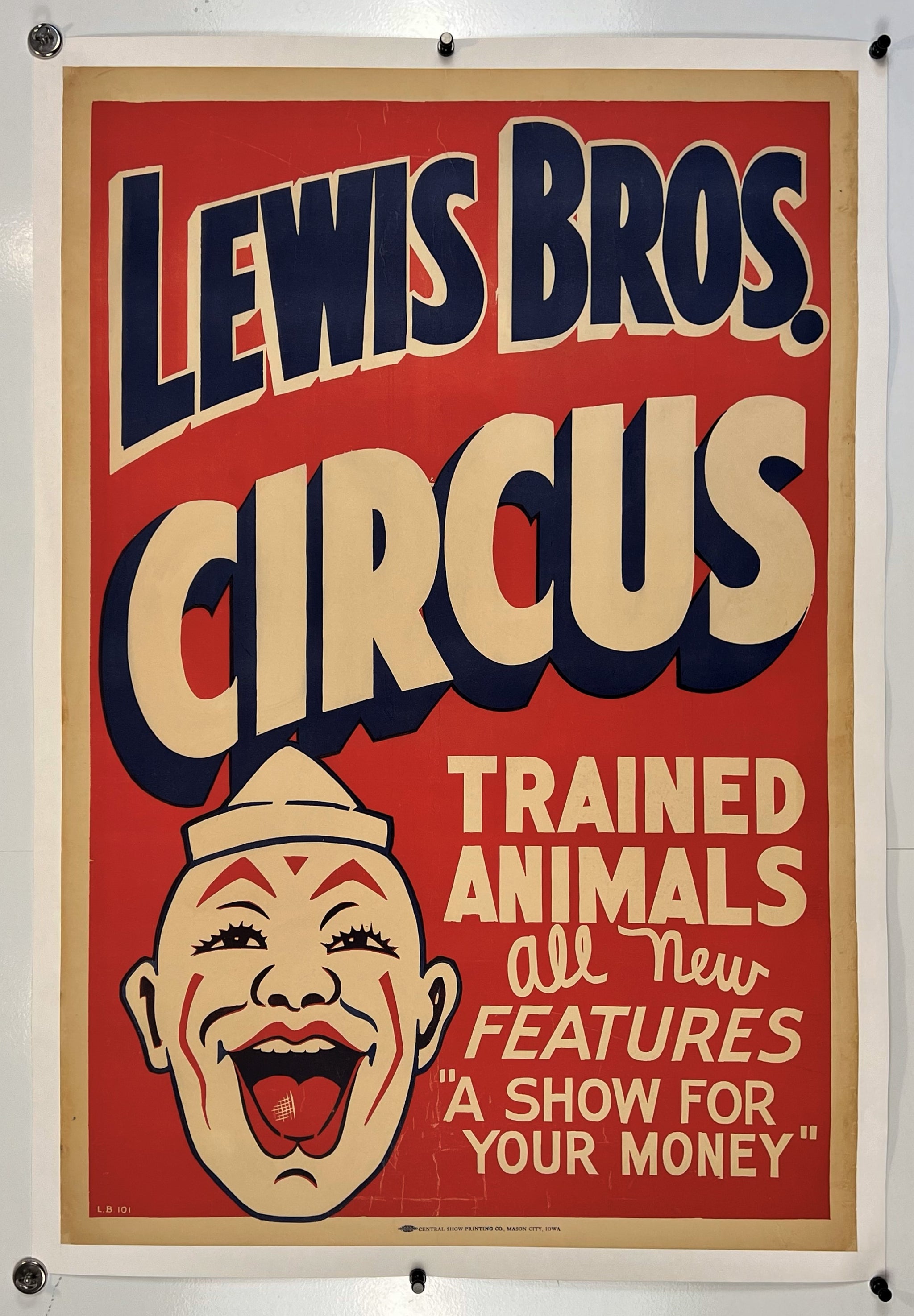The photograph captures a vintage circus poster that appears to be from the early 20th century. The poster is mounted on a white background and features a distinct design with multiple colored borders: a white outer border, followed by a light yellow-brown (or gold) inner border, and a red main background. Prominently displayed in bold blue letters, outlined in white, is the text "Lewis Bros. Circus," emphasizing the renowned Lewis Brothers Circus. Beneath this, there's a striking image of a clown, characterized by his big open red mouth, red face paint, white triangular sailor's hat, pronounced eyelashes, and a playful expression. To the right of the clown, in off-white text, the poster advertises "Trained Animals," "All New Features," and the slogan “A Show For Your Money.” The edges of the poster are secured to the wall with metal nails, three at the top and three at the bottom, further suggesting its age and authentic preservation for historical posterity.